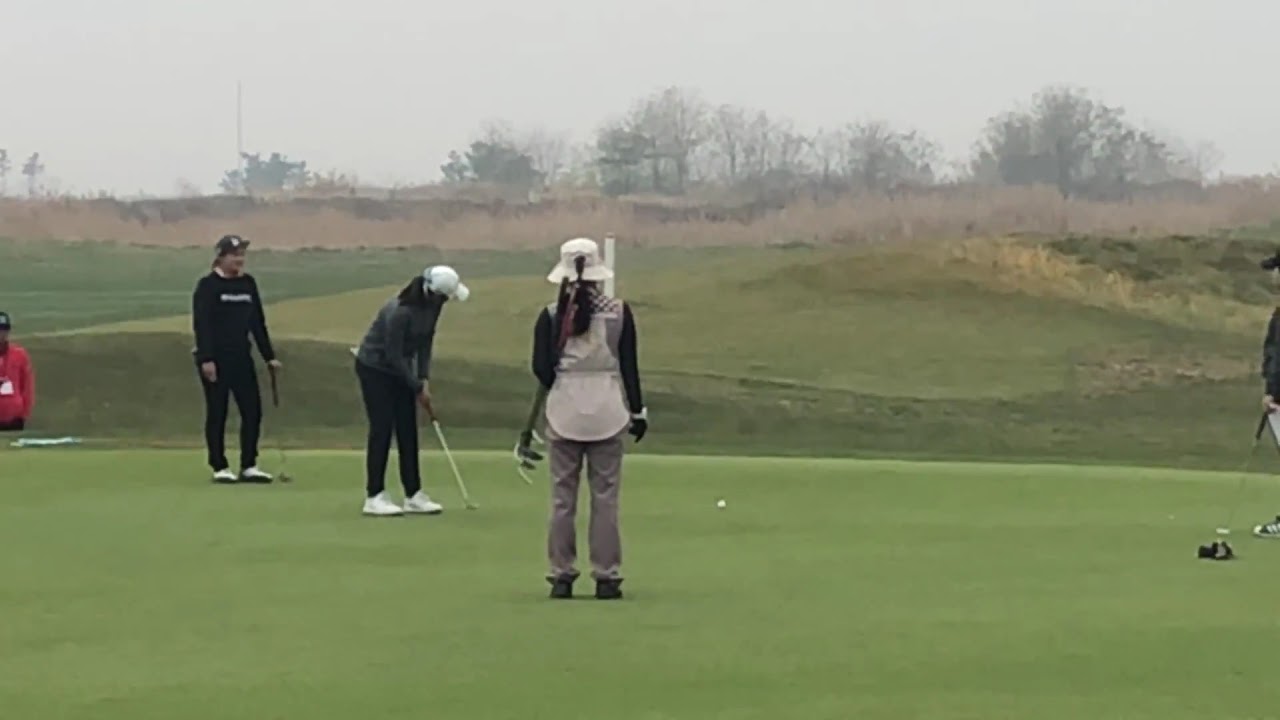This detailed photograph depicts a lively scene on a well-manicured, green golf course under a cloudy, overcast sky. The central focus is on a group of golfers, primarily women, engaged in a game. In the foreground, the grassy surface is pristine and flat, while the background transitions into a hillier, rougher terrain dotted with trees and a structure resembling a tower.

In the mid-left of the image, a golfer with long dark hair tied in a ponytail is captured mid-stroke, wearing a dark gray, long-sleeved jacket, black pants, white sneakers, and a white cap with a darker band. The white golf ball they just hit is seen rolling on the green. Another player, likely the caddy, stands nearby, identifiable by the golf clubs strapped over their back. They wear dark gray pants, a broad white hat, and dark shoes with billowed-out tops.

To the right side, another golfer, clad in khaki pants and a dark top, is visible. A spectator in red with a dark hat and pants stands slightly off to the left, observing the game. Additionally, partially obscured on the far right, there is a figure in black and light-colored pants holding a club. This dynamic composition, marked by vibrant colors including green, red, white, black, tan, gray, and purple, captures the essence of a competitive day on the golf course.